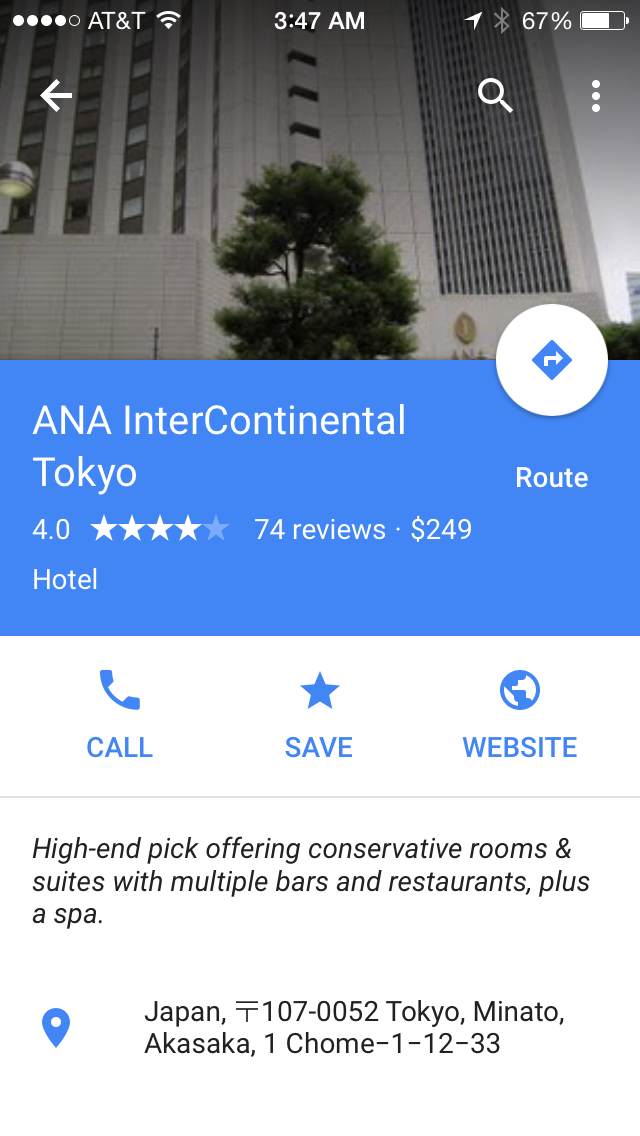This image is a screenshot taken from a Maps app on a smartphone, displaying detailed information about the Anna Intercontinental Hotel in Tokyo. 

In the upper left corner, indicators for signal strength and AT&T service, as well as Wi-Fi, are visible. At the top center of the screen, the time is shown as 3:47 AM, with all this text in white. In the upper right corner, the battery percentage, Wi-Fi, and location icons are displayed.

Central to the screen is a small image of the Anna Intercontinental Tokyo Hotel, occupying approximately 20% of the screenshot. Directly below this image, a blue information bar spans about 20% of the screen, indicating that the hotel is rated four out of five stars based on 74 reviews, with a nightly rate of $249.

Beneath the blue bar, a link offers directions or routing to the hotel from the user's current location. Further down, three interactive options are displayed: "Call" with a phone icon above it, "Save" with a star icon, and "Website" with a globe icon. 

At the bottom of the screenshot, a descriptive hotel tagline is visible, stating: "High-end pick, offering conservative rooms and suites with multiple bars and restaurants plus a spa." Finally, the hotel's address is listed below this description.